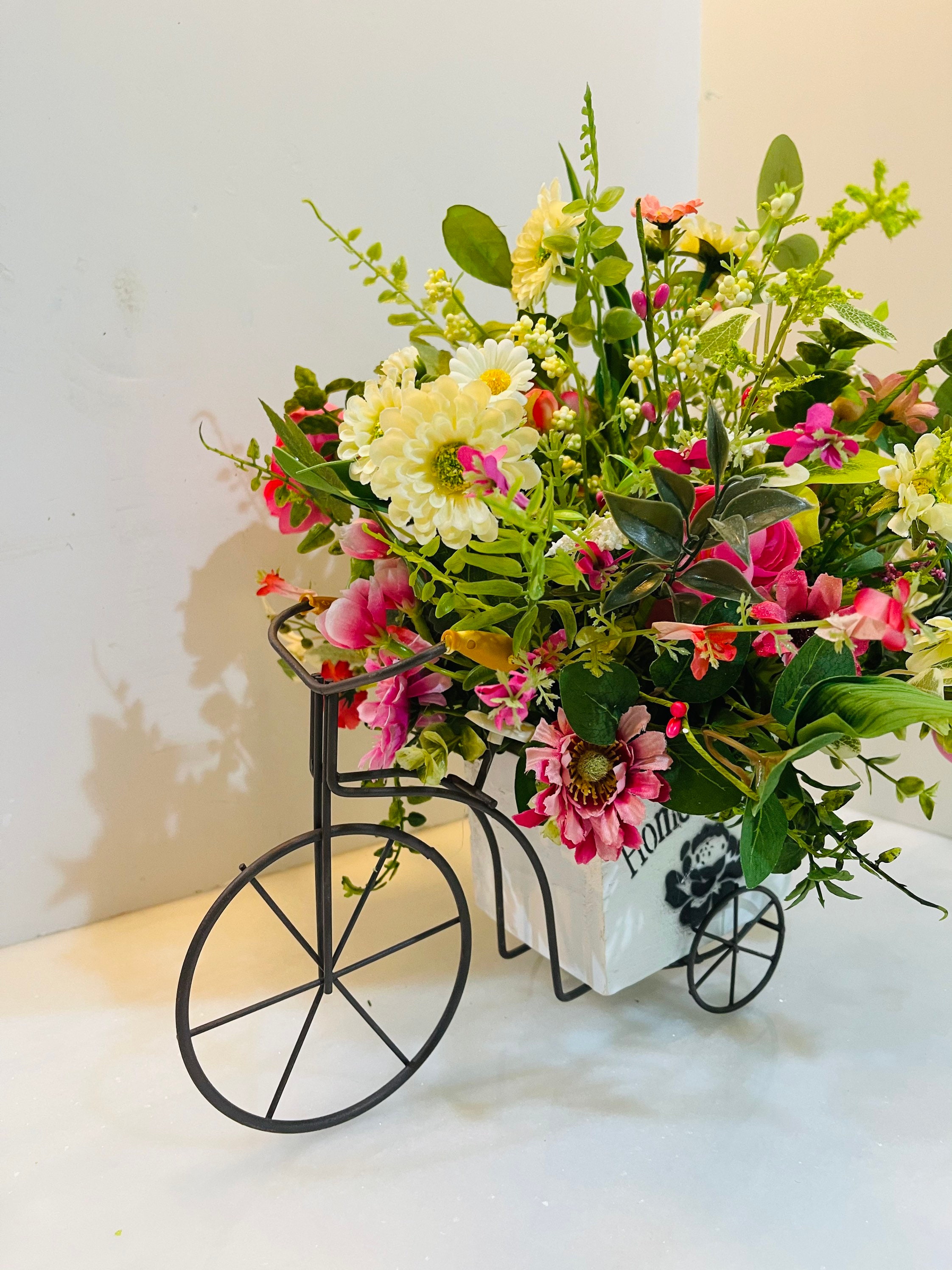The image depicts a decorative, miniature bicycle design that serves as a unique flower pot holder. The bicycle features a prominent, large front wheel and curving metal handlebars, which sweep down to a sturdy, white square base. The white vase, adorned with black designs and possibly inscriptions, sits securely on this base. This vase contains a vibrant and diverse bouquet of flowers, casting distinct shadows on the white platform and wall, hinting at a light source from the right side of the image.

Amidst the bouquet are various flowers, including daisy-like ones with either yellow petals and green centers or white petals with yellow centers. Nestled below these are numerous dark rosy pink flowers, complemented by a mix of red, yellow, and possibly purple blooms and unopened buds. Green leaves and ferns protrude and cascade from the vase, adding lush greenery to the arrangement. The scene is set against a white backdrop, where the right edge of the wall and the meeting point of the wall and floor on the left are visible, further emphasizing the composition’s elegance and charm.